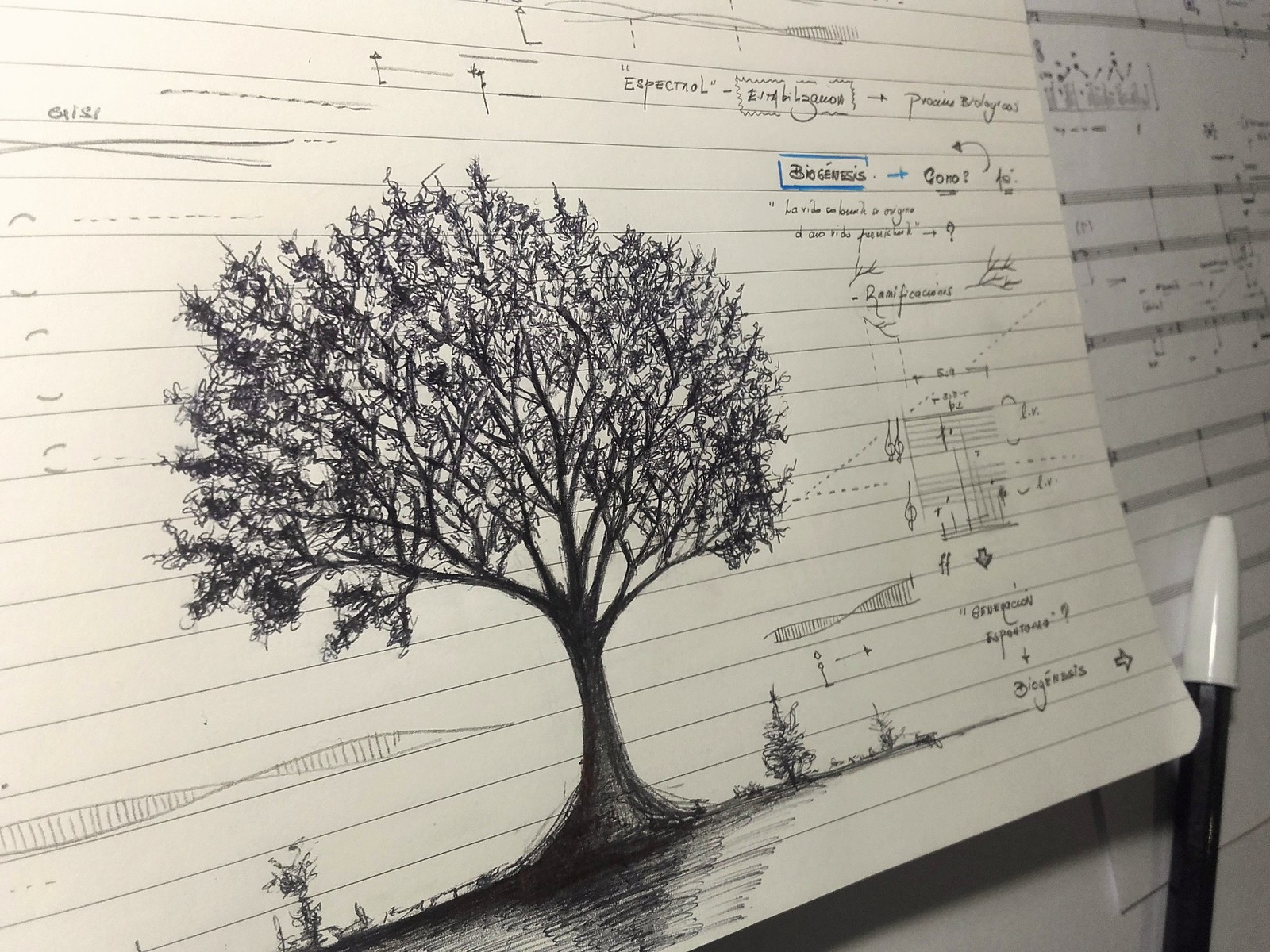The image depicts a photograph of a drawing taken from a slightly angled perspective, giving the viewer a three-dimensional sense of the scene. The photograph captures a piece of lined paper that appears to be either hanging on a wall or attached to a board. On this paper, a highly detailed tree is meticulously drawn in pen, showcasing numerous branches and leaves. The artist's skill is evident in the intricate shading of the tree and the small bushes that are thoughtfully illustrated around its base. Scattered across the paper are various writings, including references to "biogenesis" and several formulas, suggesting that the document may be related to academic or scientific work. The combination of artistic and scholarly elements creates a fascinating juxtaposition, showcasing both creative and intellectual efforts.